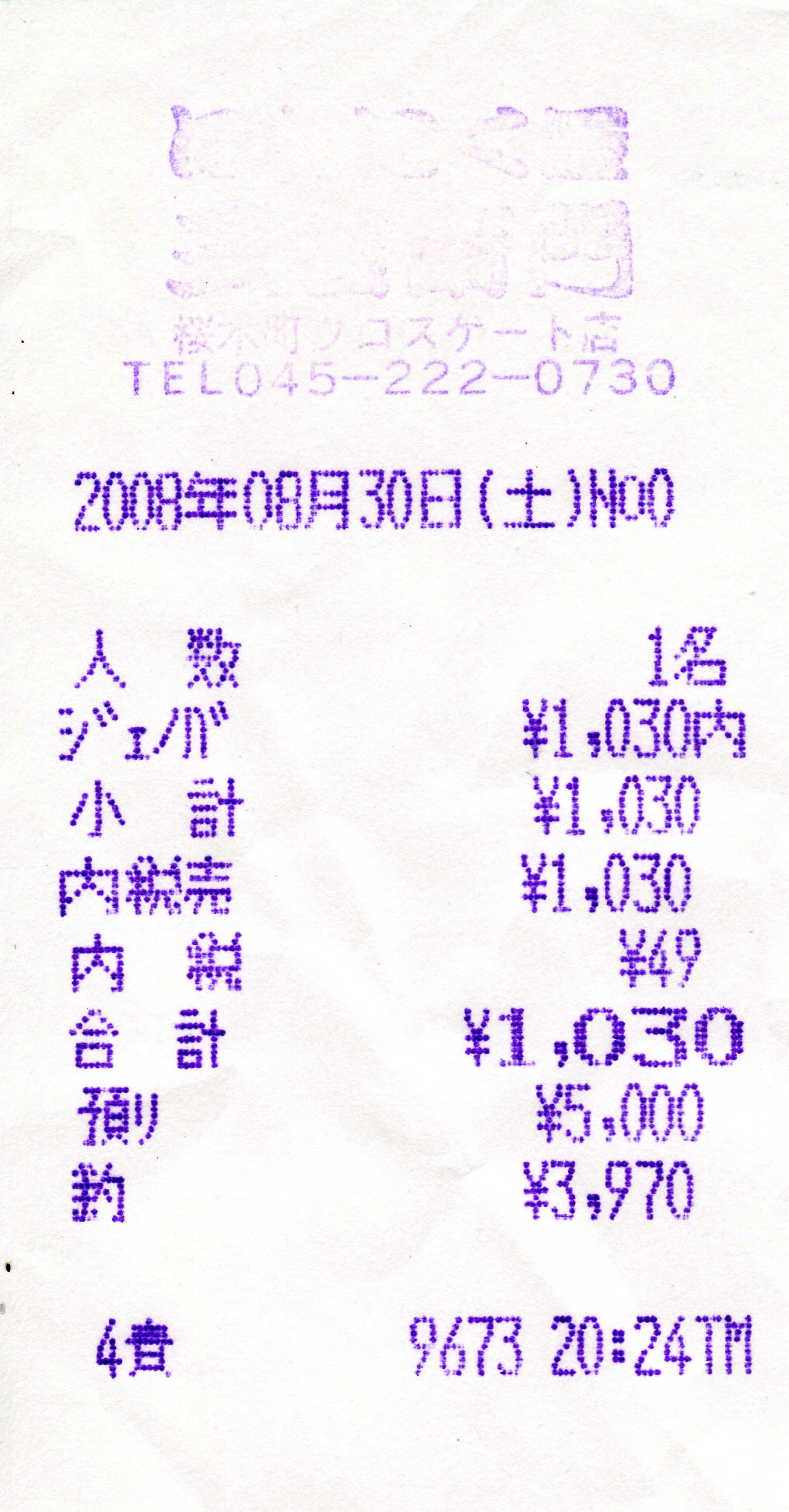This image features a white receipt with purple printing, predominantly in Japanese characters. The receipt likely pertains to a transaction involving yen, given the numerical and symbolic details. At the top, there's a faint logo and a telephone number, 045-222-0730, along with the numerals 2008 and additional characters that likely denote August 30th, 2008. The body of the receipt displays several monetary values, including repeated entries of 103.00 yen and a total of 1,030 yen. The customer seemingly paid 5,000 yen and received 3,970 yen in change. Near the bottom, there’s a timestamp, '20:24,' suggesting the time of the transaction. The entire image is framed as a vertical rectangle, with the purple, pixelated text standing out clearly against the clean white background, despite some parts being faint or washed out.